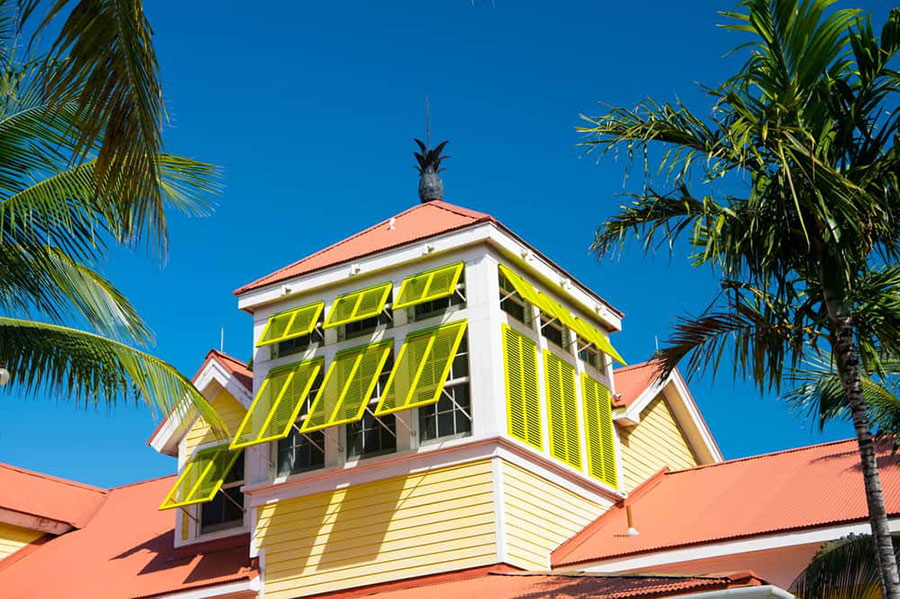The image captures the detailed top of a vibrant tropical building set against a bright blue, cloudless sky, reminiscent of a beautiful beach day. The building's roof is peach or salmon-colored and features several peaks. Central to the image is a tower-like structure with light yellow horizontal paneling and distinctive bright yellow window shutters. The shutters on the front are open, casting shadows onto the paneling below, while those on the side are closed. The white trim outlines these features, adding to the building's bright and sunny appearance. 

At the roof’s peak, a uniquely detailed black pineapple weather vane stands out vertically. Lush green palm trees frame the scene, with fronds visible on the left and a slim trunk supporting a canopy of foliage on the right. The overall scene suggests a picturesque resort building in a tropical setting.